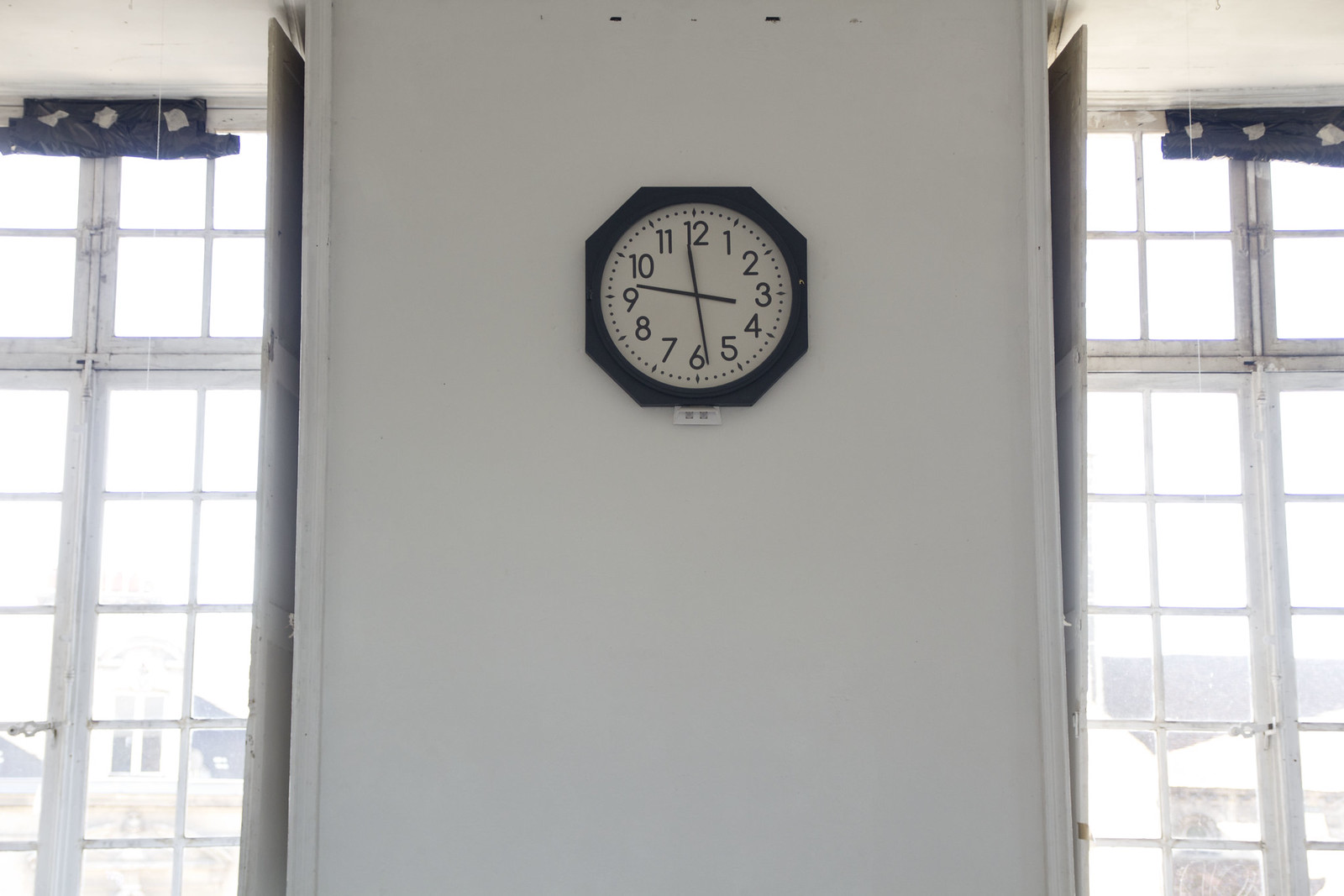The image features a white wall flanked by two double-paned windows, each adorned with white trim and a metal white-colored top edge. The windows, which open from the center, incorporate a grid pattern made of white material. Both windows are equipped with rolled-up blue curtains. Centrally positioned on the wall is an octagon-shaped black clock. The clock showcases a white circular face with black numerals from 1 to 12, accompanied by hash marks for minute increments, and black clock hands.